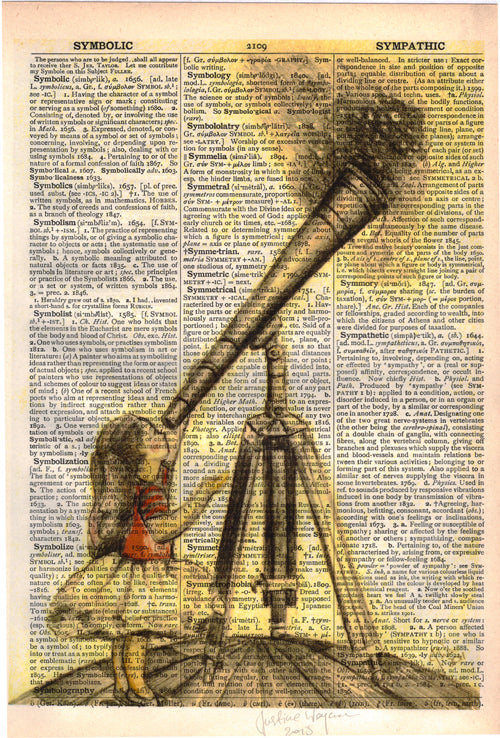In a rectangular vertical image, a young girl with long brown hair is depicted in a whimsical scene. She is wearing a red short-sleeved top paired with a fluffy white skirt. Positioned prominently in the foreground, she peers up through a large, gray telescope mounted on a tripod, which stands taller than she is. Her left arm touches the end of the telescope while her right arm reaches up into the air. The background is an intricate print that resembles an old, discolored newspaper or dictionary page with dense, minuscule text arranged in columns. Notably, among the barely readable words, the terms "symbolic" and "sympathetic" appear. Adding to the fantastical nature of the image, black smoke billows from the end of the telescope as it points towards the sky, merging the elements of a textured historical print and a vibrant, colored drawing.